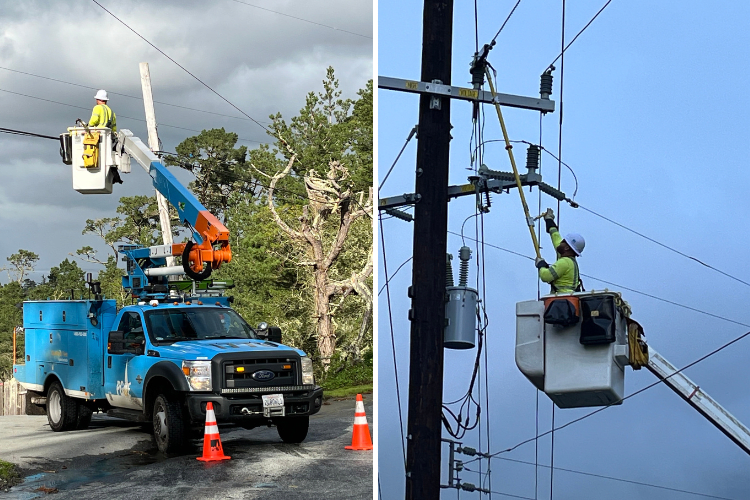The image features two side-by-side photos of utility workers performing aerial electrical maintenance. On the left, a blue work truck equipped with a multi-colored cherry picker (orange, blue, and white) is parked along a street, with safety cones placed in front. Inside the elevated cherry picker, approximately 15 feet in the air, a worker donning a yellow reflective vest and a white hardhat is positioned close to thick electrical lines. The background includes dark gray clouds and some trees. The right photo zooms in on another worker, similarly clad in a yellow reflective vest and white hardhat, standing in a white cherry picker bucket. He is manipulating electrical lines using a large, roughly 10-foot extension tool, with his left hand steadying the base and his right hand working a lever. An electrical pole is visible to the left of this worker.